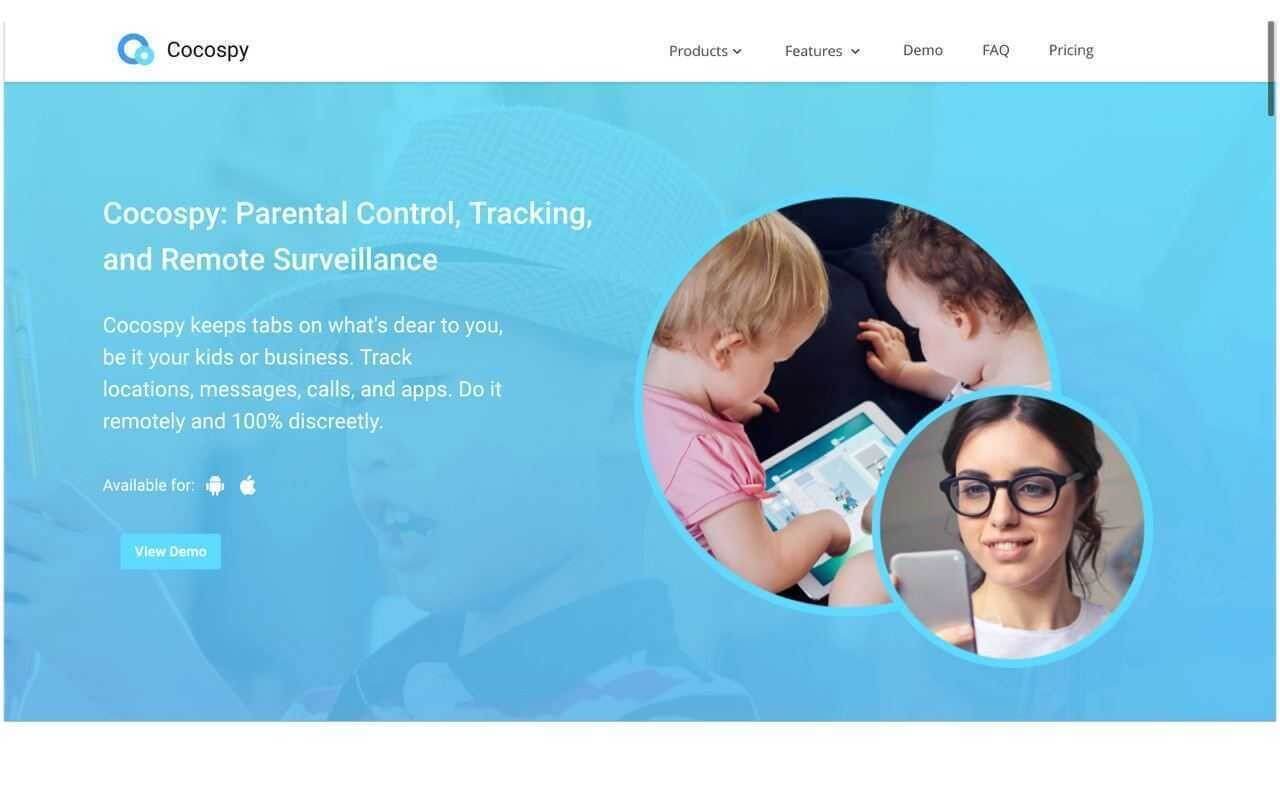Screenshot of the CocoSpy Homepage on a Desktop Browser

The screenshot displays a browser window open to the homepage of CocoSpy, a parental control, tracking, and remote surveillance service. In the top left corner, the "CocoSpy" logo is prominently featured, consisting of the service name "CocoSpy" in text, accompanied by a logo of two blue circles—a larger dark blue circle with a smaller light blue circle positioned on its lower right edge.

The navigation bar at the top of the page includes tabs labeled "Products," "Features," "Demo," "FAQ," and "Pricing." Both "Products" and "Features" have expansion arrows next to them, suggesting drop-down menus that provide additional navigation options when hovered over.

The main focus of the homepage is a large blue banner that dominates the center of the page. This banner includes two smaller circular images formatted similarly to the CocoSpy logo. The larger of these circles features an image of two children playing on a tablet, while the smaller circle shows a woman looking at her mobile phone, presumably overseeing the children.

To the left of these images, there is a detailed description of the service. It reads:
"CocoSpy, Parental Control, Tracking and Remote Surveillance. CocoSpy keeps tabs on what's dear to you, be it your kids or business. Locations, Messages, Calls, and Apps. Do it remotely and 100% discreetly. Available for," followed by the Apple and Android symbols, indicating the service's compatibility with both iOS and Android devices.

Below this text, a call-to-action button says "View Demo" in light blue, inviting users to see a demonstration of the service.